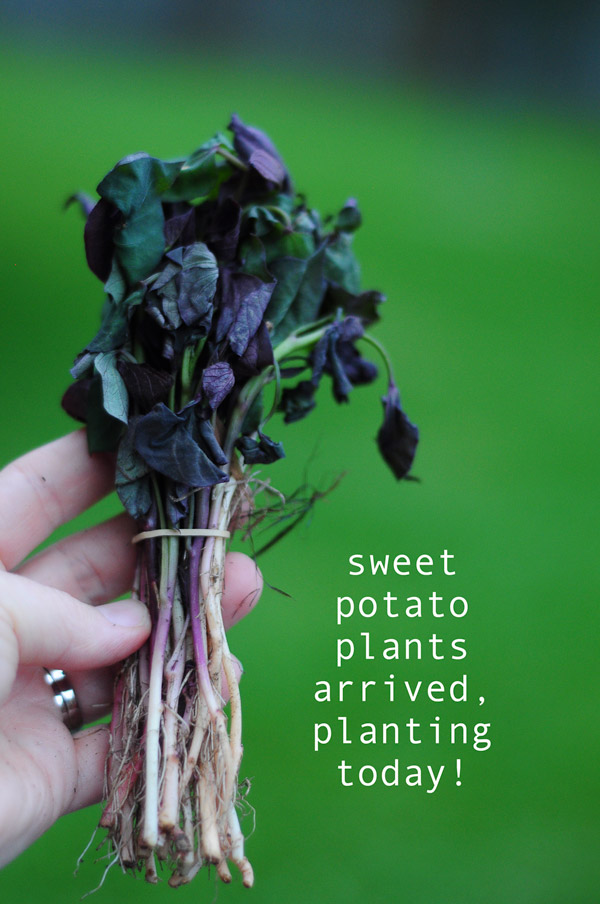A vertical photograph showcases a white hand wearing a gold ring on the left ring finger. The hand emerges from the bottom left, grasping a small bundle of sweet potato plants secured with an elastic band. These plants, with their off-white stems, sport leaves so dark they are almost black, a mix of purple and purplish-green hues. The background consists mainly of a blurred green, with subtle purplish hues diffused toward the top. In the bottom right corner, white text reads, "Sweet potato plants arrived, planting today!" This vividly detailed scene highlights the arrival and imminent planting of these tender plants.